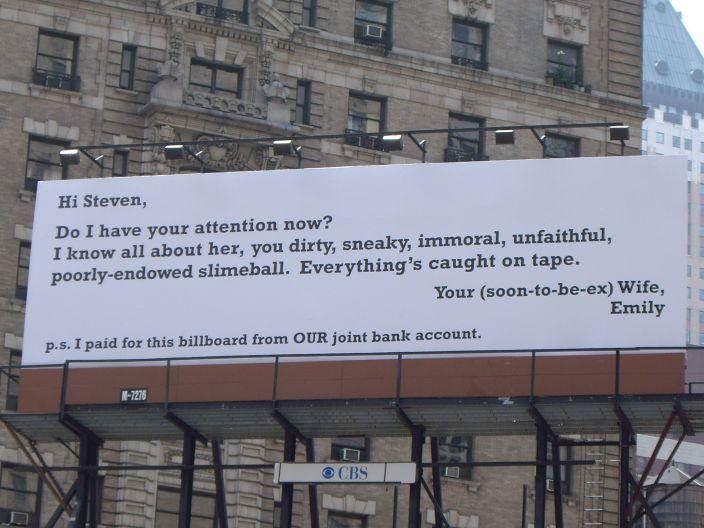In the image below, an outdoor billboard prominently stands on a black metal frame with unlit lights above it. The billboard, a horizontal rectangle, has a stark white background and bold black text reading, "Hi Stephen, Do I have your attention now? I know all about her, you dirty, sneaky, immoral, unfaithful, poorly endowed slimeball. Everything's caught on tape. Your soon-to-be ex-wife, Emily. P.S. I paid for this billboard from our joint bank account." Behind the billboard looms a large, multi-story brown brick building with numerous windows, indicating a bustling urban setting. Additionally, part of another white concrete building is visible to the right, with a clear blue sky suggesting the image was captured during daytime.